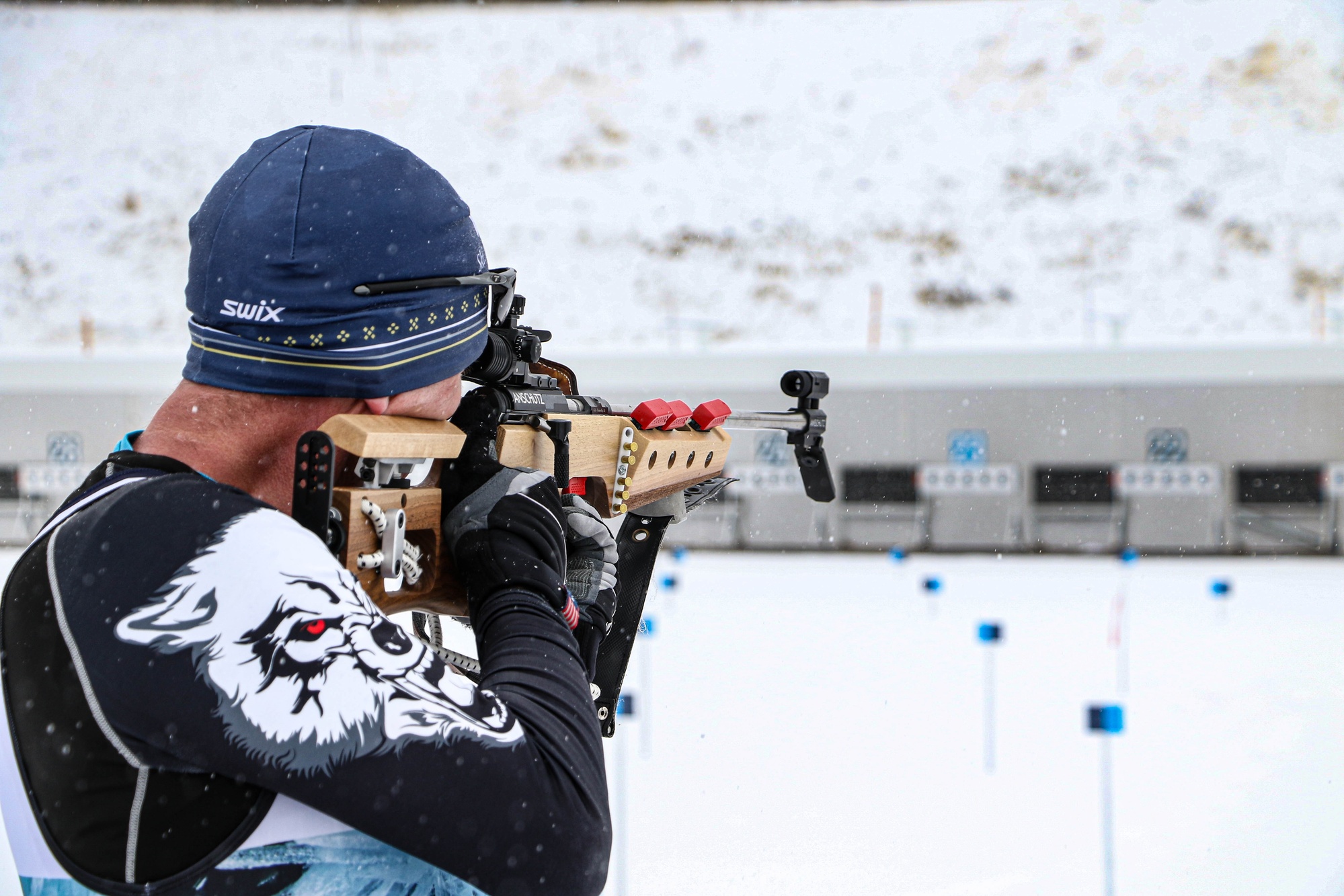The image depicts a man at a snowy outdoor shooting range, possibly participating in an alpine shooting or biathlon event. He is dressed in a long-sleeved, black, stretchy top, resembling Under Armour material, adorned with a white wolf with red eyes and large teeth near the shoulder. Over this, he wears a partially obscured white and blue uniform. He sports a blue knit beanie with tan and blue stripes and tan stars, emblazoned with the word "SWIX." His glasses are pushed up onto the top of his head. The man is aiming a light wooden rifle with red knobs and a silver piece protruding from its side. Through the scope of the rifle, a target is visible in the distance among several shooting lanes. The ground is blanketed with snow, and snowflakes are actively falling. Blue flags are planted in the snow, and targets are set up at the far end, illuminated by a blue light above.